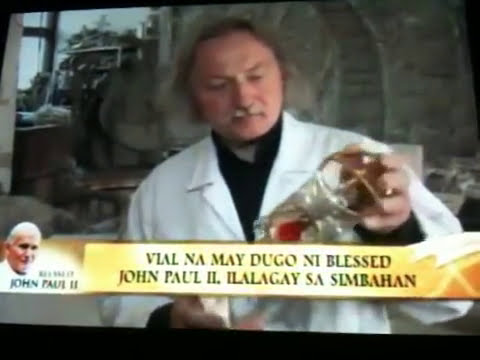A still image from a TV screen or monitor captures a gray-haired and mustached man, who appears to be a scientist or doctor, standing in an indoor setting. He wears a white lab coat over a black shirt and is intently examining a glass container held in his hand. Behind him, there is a desk area and a graphic depicting a concrete structure. At the bottom of the image, a yellow ribbon or name tag displays text in a foreign language, with part of it reading "Vyal Na Me Dogo Ni Blest Jonpol Tu Ila Lage Sa Simbahan," along with a picture of Pope John Paul II. The overall scene hints at a religious documentary or scientific video.